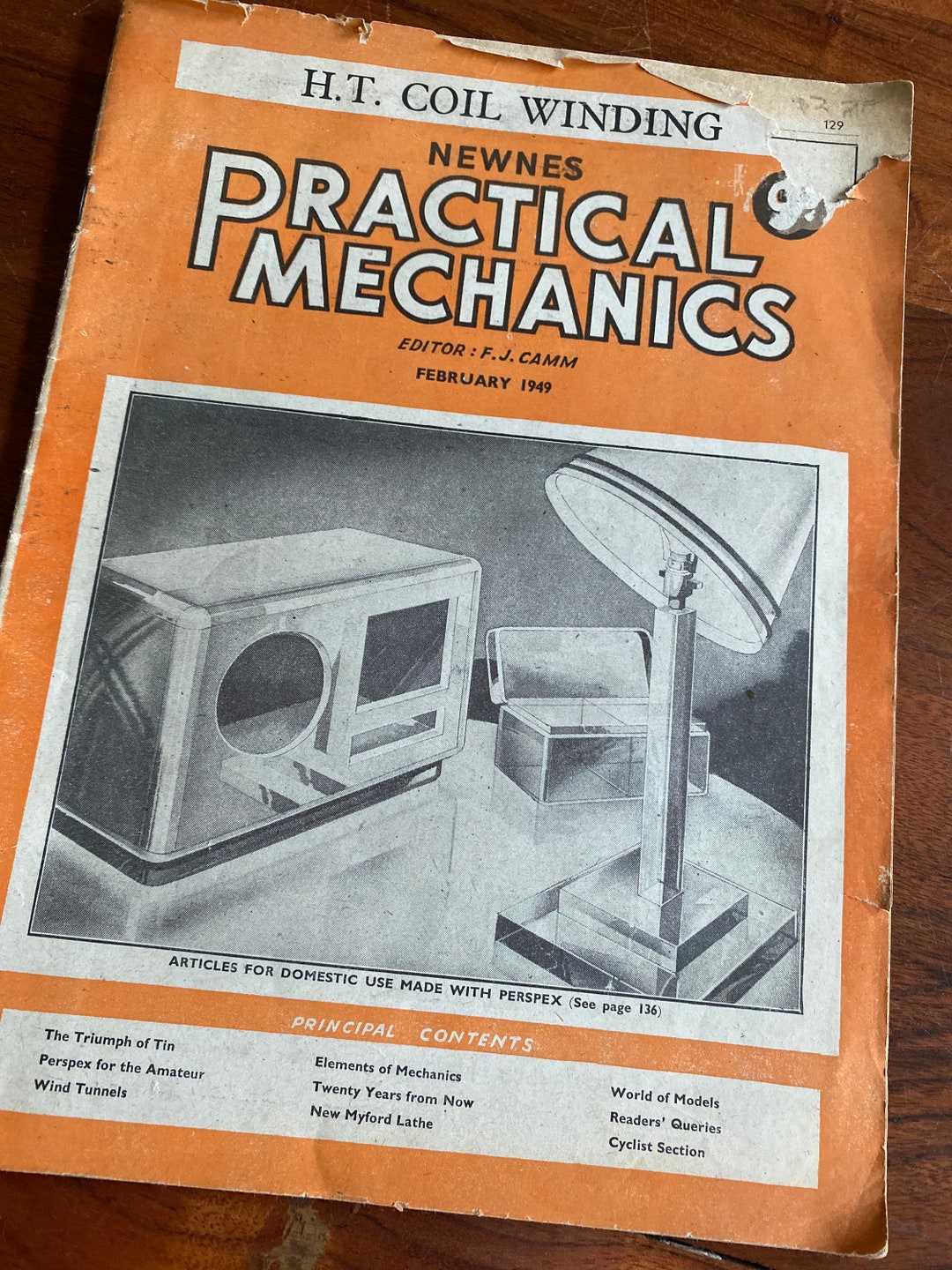This detailed photograph captures the worn and vintage front cover of the February 1949 issue of "Practical Mechanics." The magazine, edited by F.J. Camm, prominently features the headline "HT Coil Winding" in bold black letters on a white stripe across the top. Below the headline, in white text on an orange background, it mentions "Newness" and "Articles for domestic use made with Perspex," directing readers to see further details on page 136. The cover also includes a black and white photo depicting a table with a lamp and a radio, labeled in white text to indicate items made from Perspex. The bottom section lists the principal contents of the magazine in three columns, including "The Triumph of Tin," "Perspex for the Amateur," "Wind Tunnels," "Elements of Mechanics," "20 Years from Now," "New Myford Lathe," "World of Models," "Reader's Queries," and "Cyclist's Section." The cover shows signs of age, such as tears at the top, a pencil-written price of $2.70, and overall wear. The entire composition renders a nostalgic glimpse into mid-century mechanical interests and innovations.